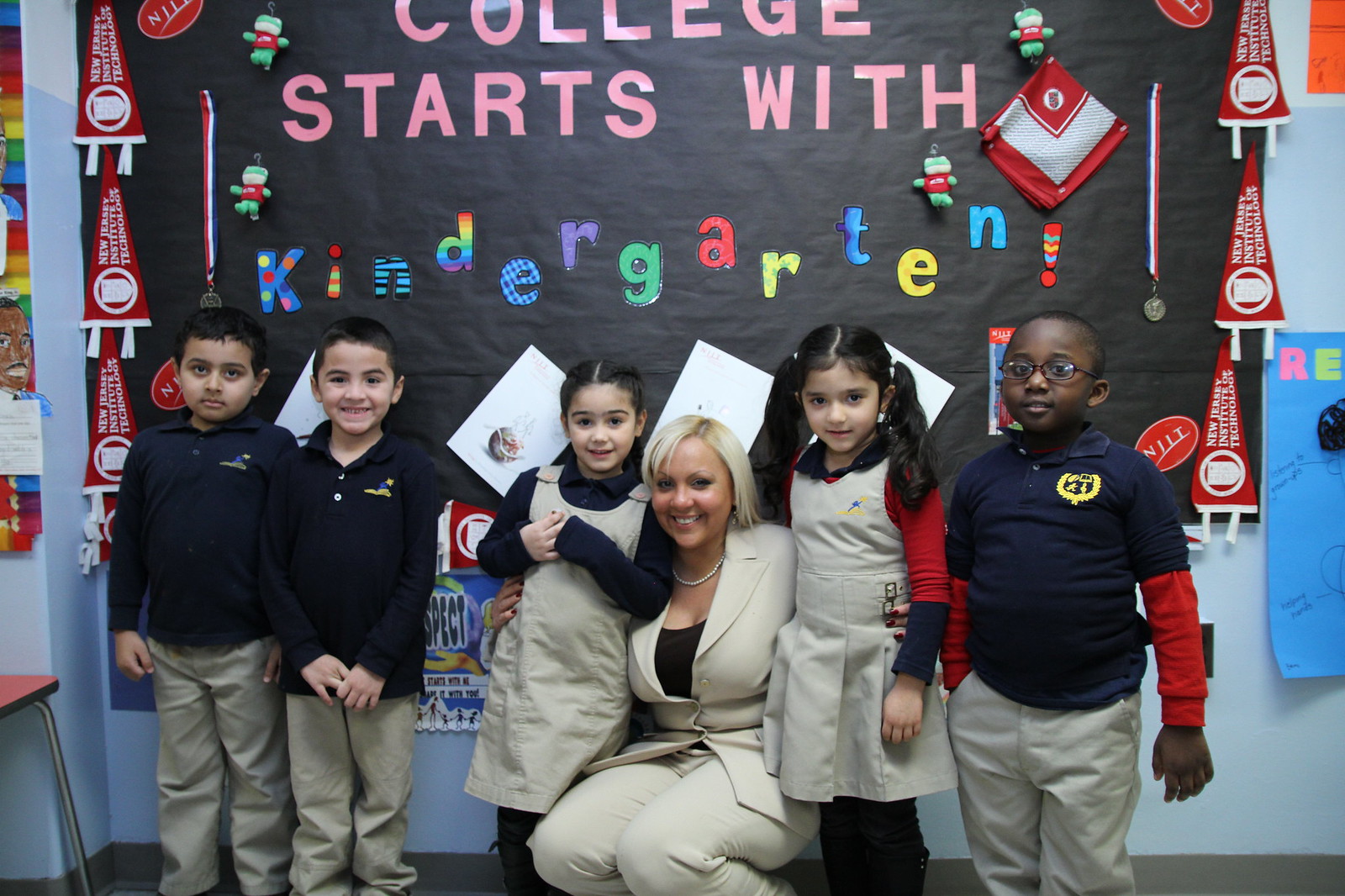This charming picture captures a kindergarten class, likely from a private school in New Jersey. The image features six people: five young children and a teacher. The children, three boys and two girls, are all smiling and dressed in uniforms. The boys are sporting navy blue shirts with either gray or khaki-colored pants. One boy, on the far left, wears a navy blue short-sleeved shirt with a yellow emblem. The two girls wear gray or khaki-colored dresses paired with navy blue shirts. The girl with pigtails is distinguished by a red shirt worn over her navy blue shirt.

The teacher, who is in the center, is a blonde woman wearing a white pantsuit with a black shirt. She has her arms affectionately around the two little girls, adding a nurturing touch to the scene. Behind them, a sign crafted with evident care reads, "College starts with Kindergarten," emphasizing the importance of early education.

The background includes various articles and artifacts, such as a banner for the New Jersey Institute of Technology, which suggests the photo was taken in New Jersey. Also visible are medals, flags, and colorful decorations adding to the festive, celebratory atmosphere. The bright, cheerful environment, paired with the smiling faces, suggests this could be a pre-graduation picture. The photograph captures a moment of joy and achievement for this young class, taken by an external observer.